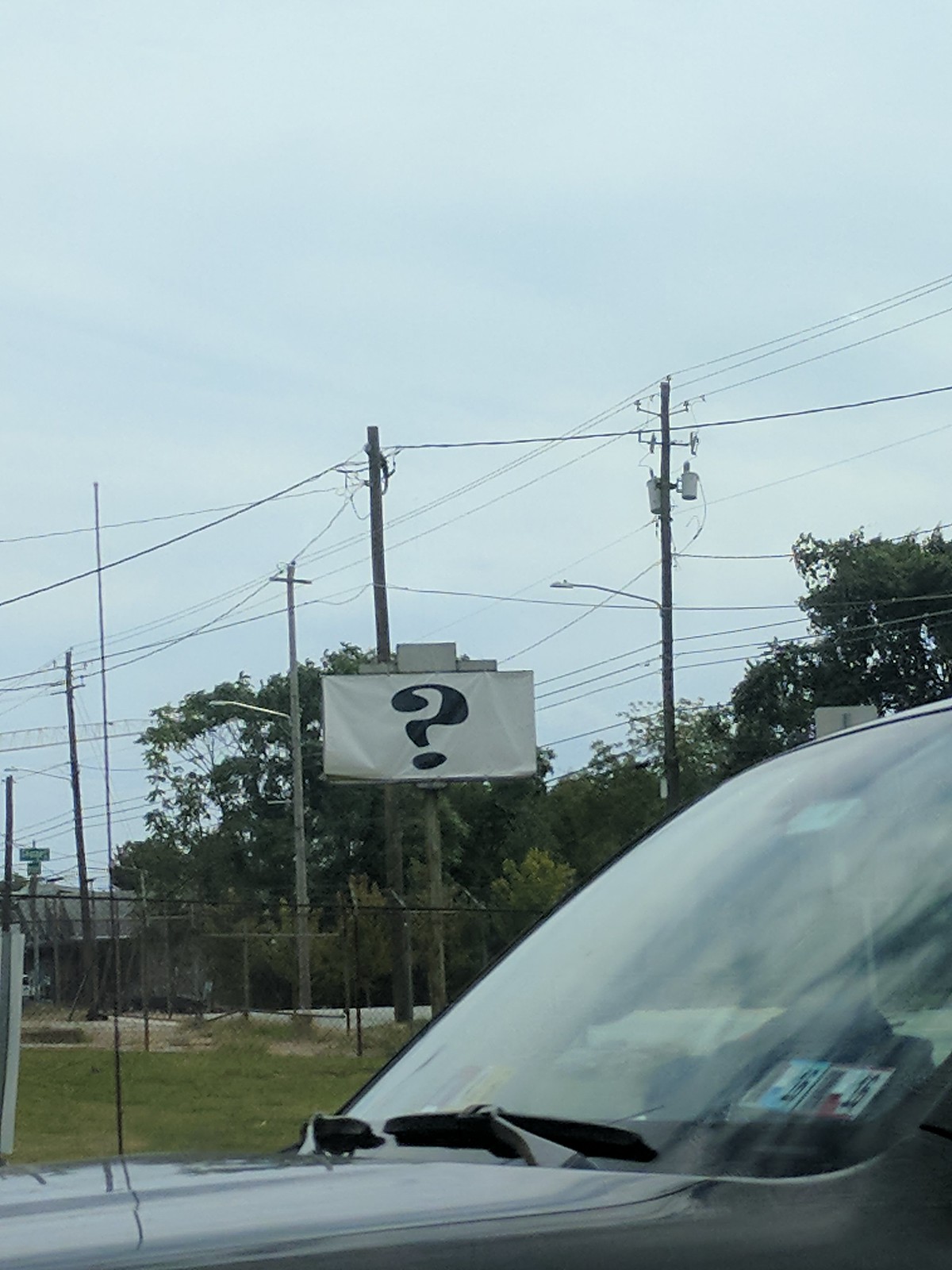This color photograph taken outdoors captures a daytime scene dominated by a large, enigmatic billboard displaying only a black question mark on a stark white background. The billboard, set against a blue sky with wisps of clouds, is framed in the background beyond a vehicle's windshield, which occupies the lower foreground of the image. The car, appearing to be dark in color, partially reveals its hood and windshield wipers, adding a layer of urban context. 

Electric and telephone poles with wires stretch horizontally across the frame, intersecting a patch of green grass and a chain-link fence. The scattered poles serve as accents leading the eye towards the mysterious billboard. A few green trees rise from the right side of the image, extending towards the left, merging with the photograph's distant elements. A barely discernible street sign occupies the left center, adding to the layered visual hierarchy. Overall, this peculiar yet intriguing image combines elements of the mundane and the mysterious, evoking a sense of curiosity and urban grit.